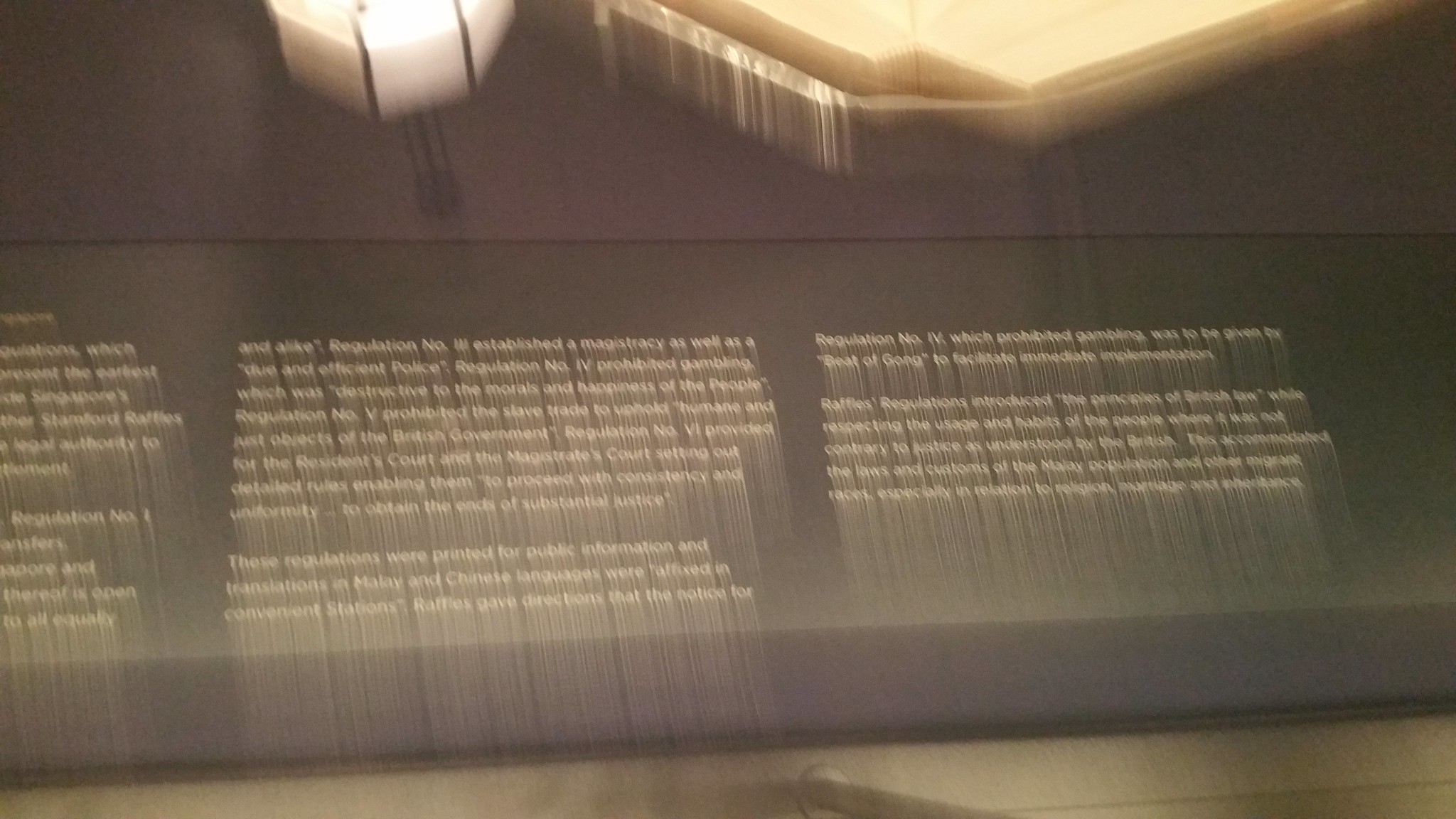This image captures a blurry photograph of an informational placard typically found in a museum or zoo setting. The placard features white text set against a black background, providing detailed descriptions related to the exhibit. The display is framed by a prominent purple border at the bottom, with additional purple accents above. Natural and artificial light sources create a mixed lighting effect; one source appears from an opening above and to the right, casting a diffuse glow, while another light source seems to emanate from the left, aimed upwards. These lights contribute to the overall blurred ambiance of the scene. The floor beneath the display is composed of gray granite tiles, adding to the structured environment. Shadows suggest the presence of onlookers, indicating that someone is standing nearby, possibly examining the exhibit.